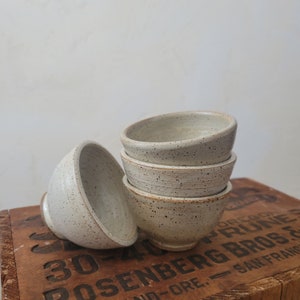This color photograph showcases a meticulously arranged scene featuring four ceramic bowls on a wooden crate with a rustic aesthetic. The focal point is a stack of three identical, grey-colored bowls with delicate black speckles, indicative of pottery craftsmanship. Adjacent to the stack lies a single bowl, tilted on its side with the open end facing the stacked bowls. The bowls rest upon a wooden crate that displays partially obscured text, including phrases such as "BOSSENBURG BROS" and "30-40 PRUNES," hinting at a historical or commercial context. The background is a subtle grey, complementing the overall muted color palette and adding to the serene composition of the square-framed photograph.